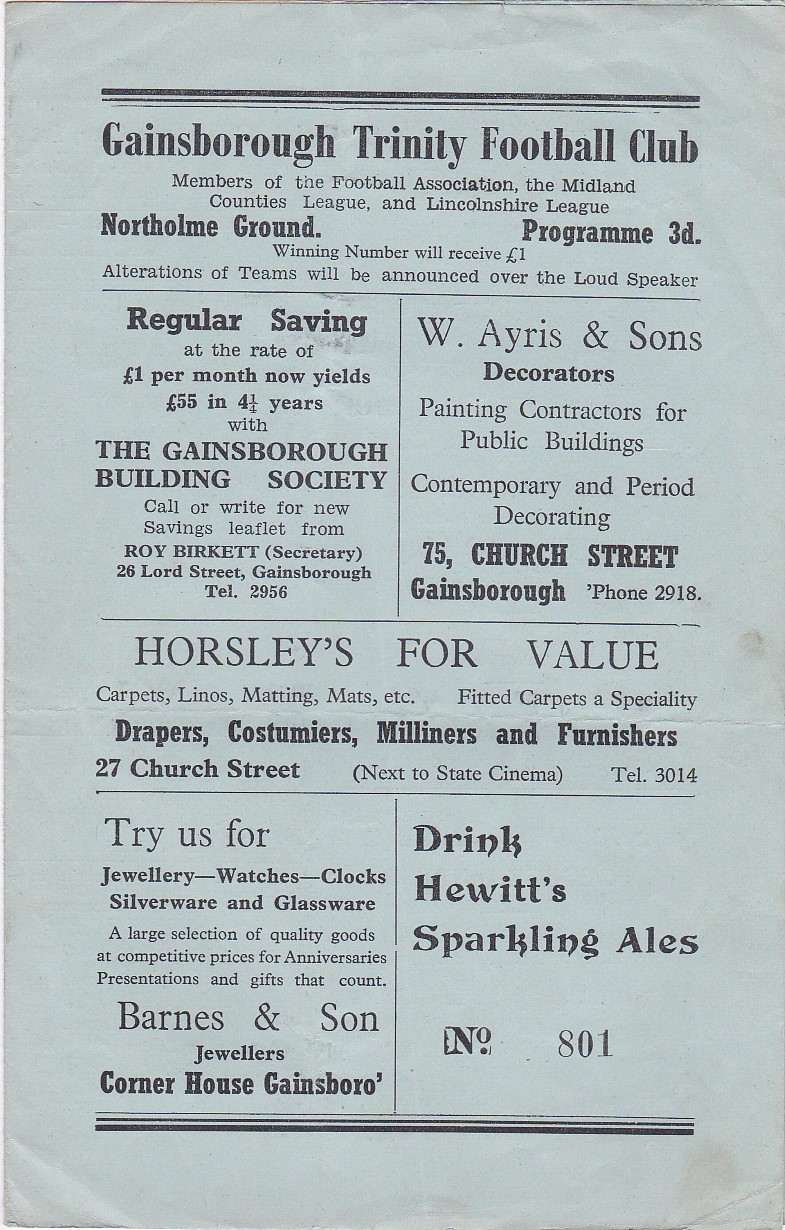This image showcases a page from an old vintage football program, likely from the Gainsborough Trinity Football Club. The program, printed on light blue paper, primarily features black text in varying fonts that resemble a Times New Roman typewriter style. Across the top, it prominently reads "Gainsborough Trinity Football Club" and identifies the club as members of the Football Association, the Midland Counties League, and the Lincolnshire League. Below, it states “Northolme Ground Program 3D,” indicating the price, and mentions that the winning number will receive one pound. Alterations to teams would be announced over the loudspeaker.

The lower half of the page is filled with advertisements. These include promotional content from the Gainsborough Building Society, highlighting a regular saving plan of one pound per month yielding 55 pounds in four and a half years. Another ad from W Iris and Son, decorators and painting contractors, provides details about their services for public buildings and contemporary period decorating, located at 75 Church Street, Gainsborough. Additional advertisers include Horses for Value, offering draperies, cosmetics, millers, and furnishings; Barnes and Son Jewelers, specializing in jewelry, watches, clocks, silverware, and glassware located at Corner House, Gainsborough; and Drake Hewitt’s Sparkling Ales, noted with the number 801. The layout and varied advertisers hint at a rich local community engaged in supporting the football club.